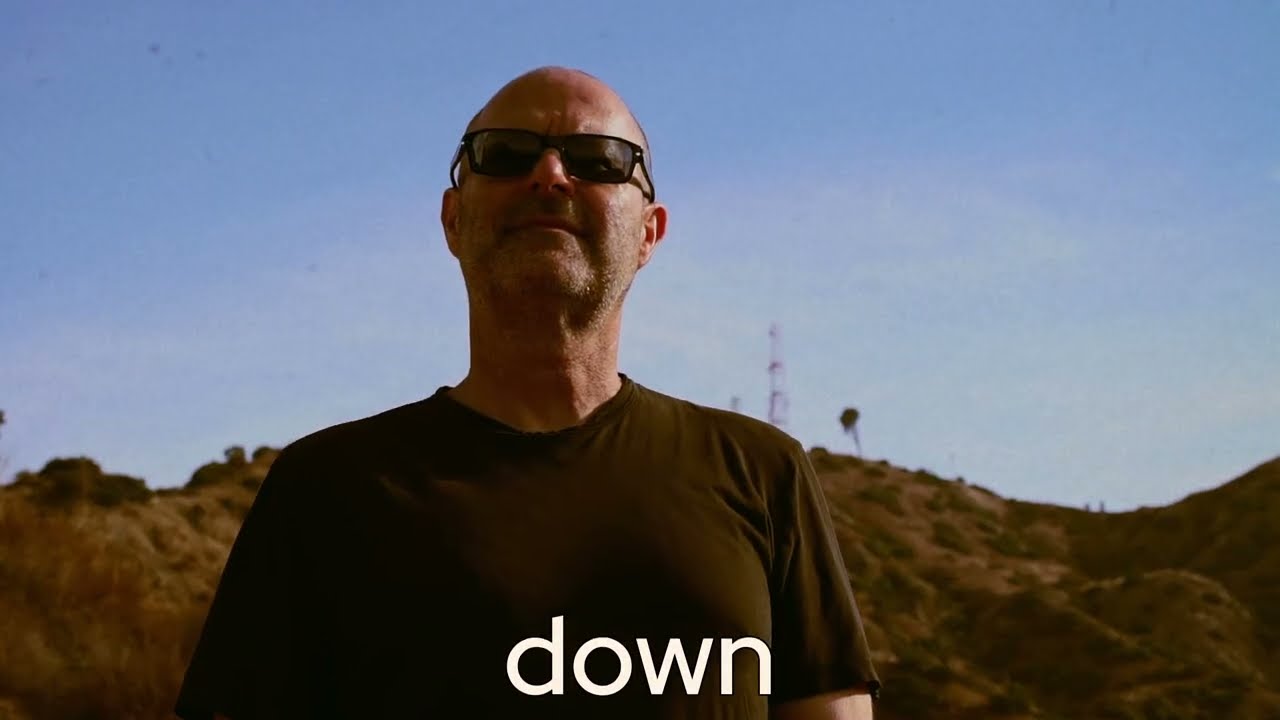The image features a middle-aged, bald Caucasian man wearing black sunglasses and a loose-fitted black t-shirt with the word "down" written in lowercase white letters at the bottom center. He has a gray stubble beard and a narrow chin. The man is centered just slightly to the left, with the sun illuminating the left side of his face. Behind him, the scene is a desolate, rocky hillscape with sparse vegetation—a mix of tiny shrubs and sagebrush—under a clear blue sky. A tower or antenna station is visible over his left shoulder, adding to the rugged outdoor setting. The photograph, likely taken with a phone or DSLR camera, captures the man's silhouette against this sun-drenched, natural backdrop, giving it an intimate and solitary feel.